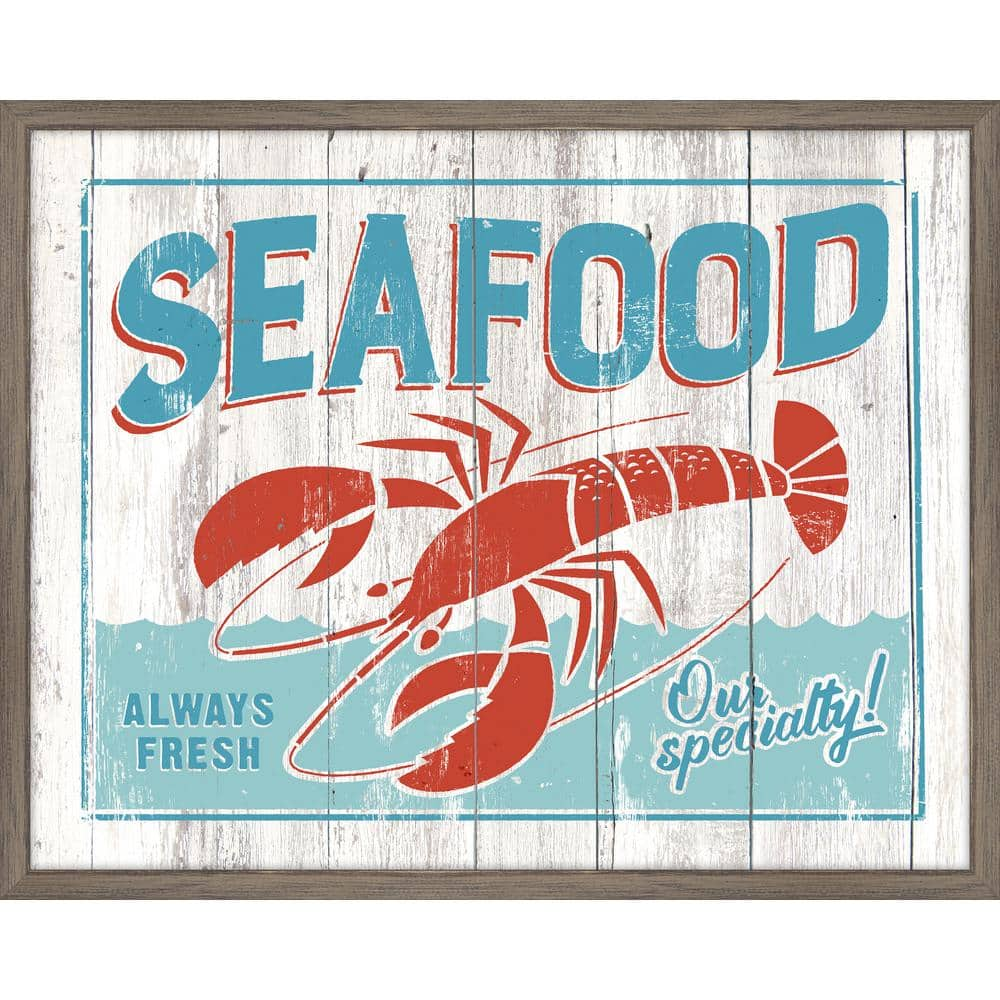This landscape-oriented color photograph captures a vintage-style sign advertising a seafood restaurant. The sign is framed in dark gray wood, which surrounds vertical whitewashed wood planks. Inside the frame, an aqua-colored border delineates the main content area. Dominating the top portion are large, aqua letters spelling "SEAFOOD," each letter accented with a red outline. Positioned just below, a detailed red illustration of a lobster, complete with claws, legs, tail, fins, and antennae, draws the eye. Beneath the lobster, the phrase "always fresh" appears in dark blue letters on the left side, while "our specialty!" in cursive script is displayed on the right. The lower third of the image features a subtle representation of blue wavy water, blending into the background and adding a touch of realism to the composition. This meticulously crafted sign blends artistic elements with a clear message, epitomizing the essence of a classic seafood eatery.